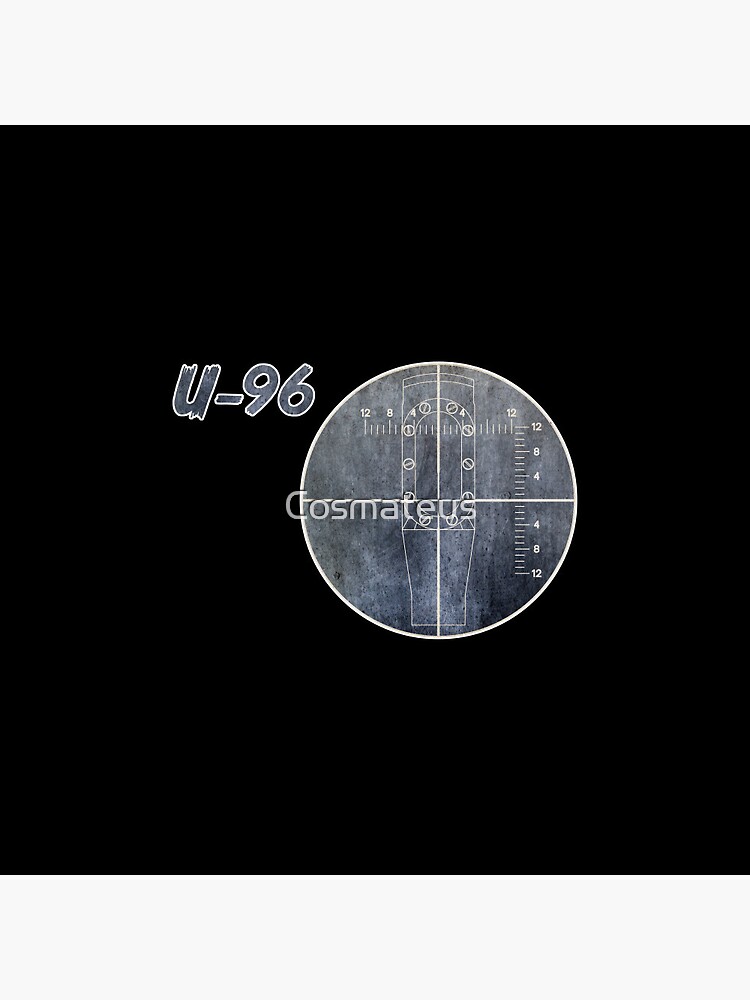The image features a simple, yet structured design set against a plain black background. Centrally aligned within the image are two main elements. To the left, there is a stylized inscription of "U-96," featuring a lowercase "u" and a white border around the gray figures, possibly suggesting a reference to a submarine or an atomic element. Adjacent to this inscription, on the right, is a prominent gray circle outlined with a thin white line, resembling a crosshair. This circle contains intricate, superimposed designs: a gray, metallic-like material etched with calibration scales. Specifically, the vertical scale runs from 0 to 10 and is notched at intervals, whereas the horizontal scale mirrors this pattern. Within this circle, there is a rectangle with an elongated bottom, possibly resembling a neck of a guitar or some instrumentation device, marked by numerosities of 12, 8, 4, and 4, 8, 12 that align vertically and horizontally. Overlapping these details, the word "Cosmateus" (C-O-S-M-A-T-E-U-S), predominantly in lowercase except for the initial "C," is etched into the gray surface, adding an enigmatic touch to this technical and abstract rendering.